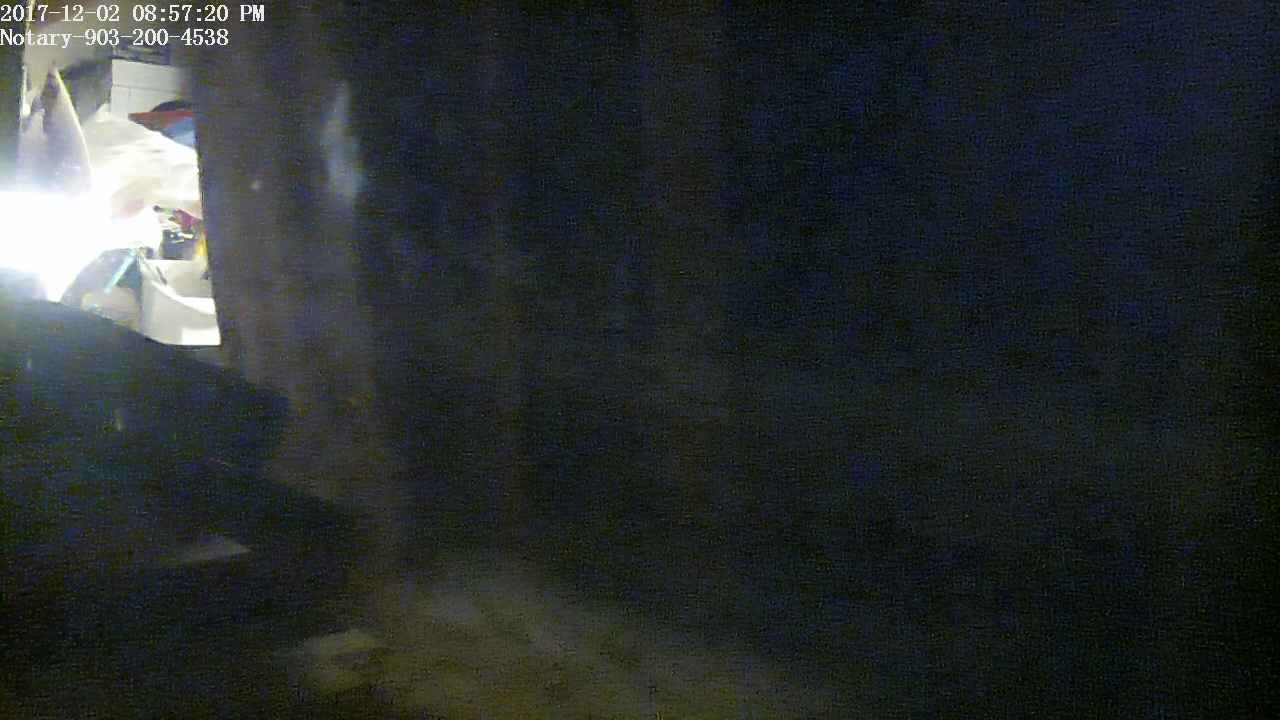In this image, a dimly lit room is captured with an overall blue and black color palette that creates a somber atmosphere. The timestamp in the upper left corner reads "2017-1202 at 08:57:20 PM," accompanied by the notation "Notary 903-245-38." Scattered across the floor are various unidentifiable piles, adding to the room's disorganized appearance. Through the window, fragments of the outside world are visible, including a white concrete surface, several white round objects, a black can, and a smaller can, lending small hints of light to the otherwise dark scene.